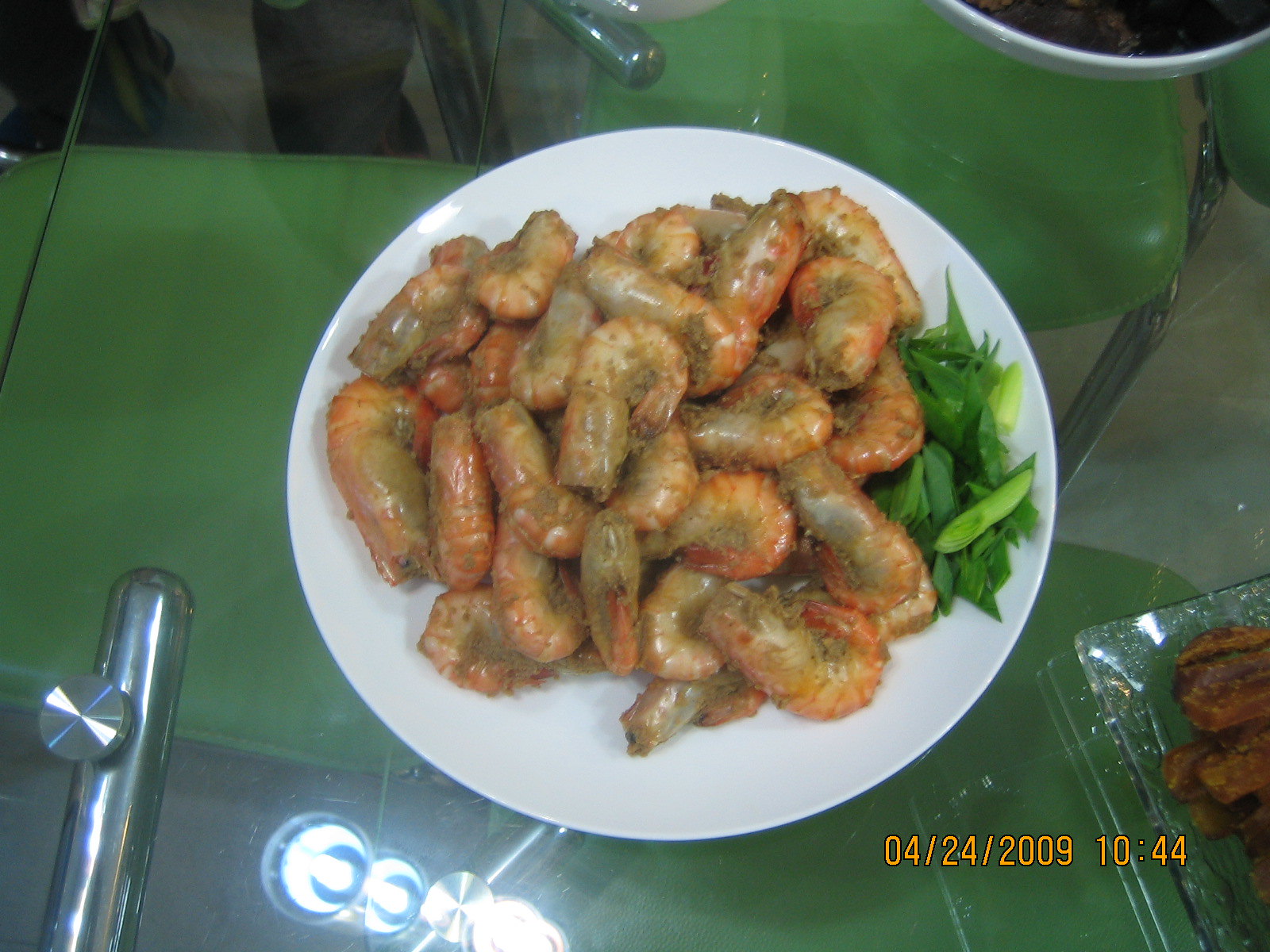This photograph captures a white circular plate piled high with headless shrimp, which still have their shells on and exhibit a tan and reddish hue. The dish is garnished with spring greens or onions on the side. The plate rests on a glass tabletop, reflecting overhead lights and supported by a visible steel or chrome base. In the background, there's a date and timestamp reading "04-24-2009 10:44." A person in gray slacks is partially visible on the other side of the table, though their posture is unclear. To the upper right of the main dish lies a bowl containing a white liquid, while the lower right features a clear glass dish with a long, brown item. The combination of elements and the setting evoke the ambiance of traditional Chinese cuisine or hot pot dining.